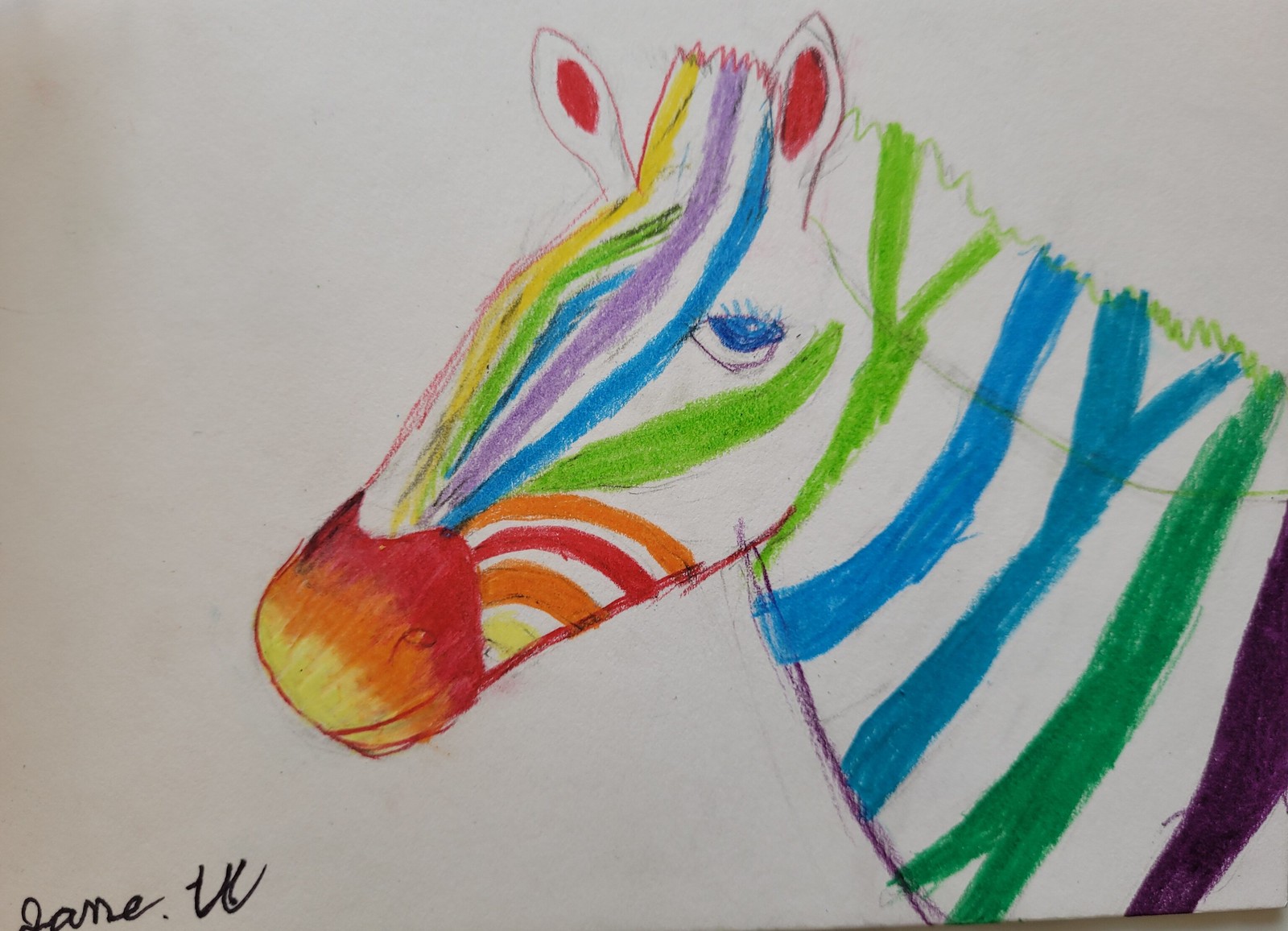This photograph features a white piece of paper, dominating the entire frame except for a small sliver in the lower right corner that reveals the brown surface beneath. The paper's lower left corner bears a barely legible artist’s signature in black paint. Central to the image is a pencil drawing of a zebra in profile, facing left and casting a side-eye glance towards the viewer. Uniquely, this zebra boasts vibrant, rainbow-colored stripes—orange, blue, red, yellow, and green—contrasting with a striking blue eye. The overall aesthetic suggests the artwork may have been created by a child.